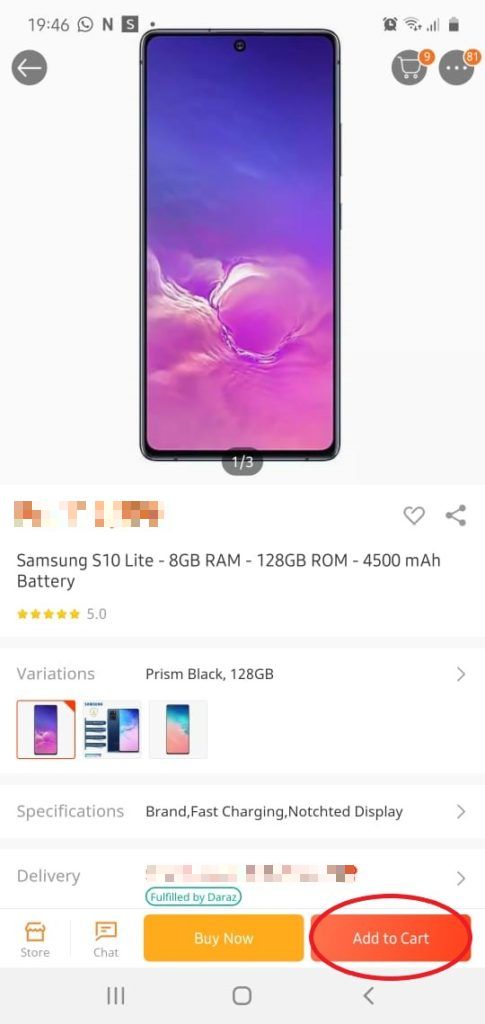The screenshot depicts a shopping interface on a smartphone. The screen is divided into two sections: the top half features a light gray background, and the bottom half shows a white background. 

In the top left corner, a black circle displays the time, with various icons adjacent to it: a black square with a white "S" icon, a battery icon, an internet signal icon showing three out of four bars, a Wi-Fi icon also showing three out of four bars, and an alarm clock icon.

Prominently, there is a large gray circle with three white dots arranged horizontally. In its top right corner, an orange circle features the number "81" in white. To the left, a green circle has a white cart icon, and further right, another orange circle contains the number "9" in white.

Below the icons, the central portion of the screen showcases an image of a smartphone with a gray border. The upper half of the phone's display appears as a blue sky, while the lower half exhibits a blend of purplish and pinkish hues, resembling water.

Under the time display, on the left, there is a small gray square with a white left arrow. Directly beneath this, within the white-background section, a portion of the screen is blurred in the left corner. To the right, there are icons for a heart outline and a share option, both in black.

The product details feature black text, describing "Samsung S10 Lite - 8GB RAM - 128GB ROM - 4500mAh battery." Directly below, a five-star rating is displayed. The text also notes variations, indicating a model in Prism Black with 128GB storage.

Additionally, there are three clickable images of phones to provide more views, and a section labeled "Specifications" with details such as the brand, fast charging capability, and matching notifications.

At the bottom right corner, a red tab with white text reads "Add to Cart," circled in red for emphasis. Next to it, a yellow tab with white text indicates "Buy Now."